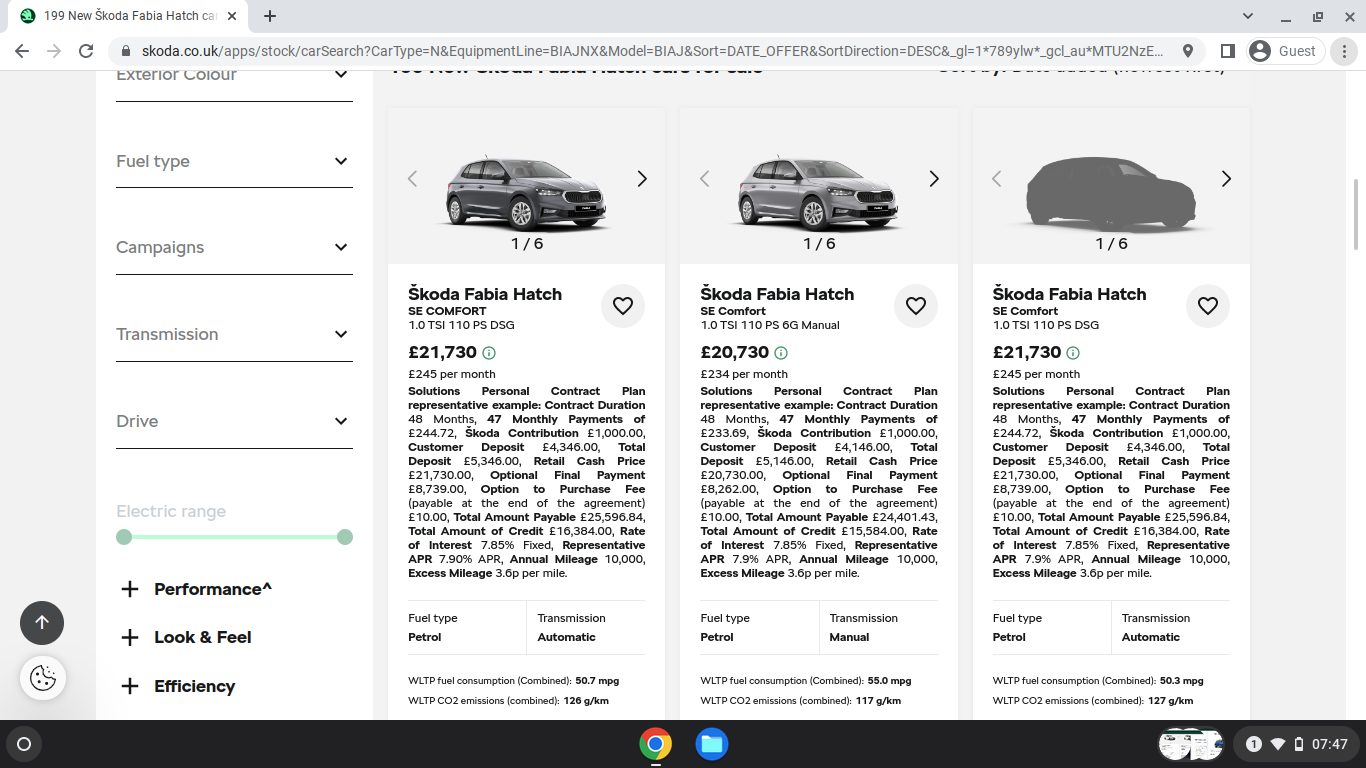This image depicts a web page from SCOTA, a car company in the United Kingdom, visible at the web address scota.co.uk. The page in focus is the car search results page. At the top left corner on a white background is the header text "199 New SCOTA Fabia Hatch Car". Adjacent to this, and to the right, runs a long gray ribbon.

Beneath the address bar, the primary content of the page is set against a light gray background. On the left-hand margin, there is a wide white vertical ribbon featuring various filtering options. These filters include car color, fuel type, campaigns, transmission, drive, with an option for electric range at the bottom that is grayed out. Below these filters, in bold dark black text, are categories labeled performance, look and feel, and efficiency, each accompanied by a black plus sign to their left.

The main content area to the right features three different car options. Each car option includes:

1. An image of the vehicle at the top.
2. The name of the vehicle below the image.
3. The price of the vehicle.
4. A brief descriptive paragraph about the vehicle.
5. Information on fuel type and transmission—specifically, petrol and automatic for the first car, a SCOTA Fabia Hatch.

At the very bottom of the screen, a black ribbon spans the entire width of the page, providing a visual boundary.

This detailed layout ensures a convenient user experience by highlighting the car options and allowing easy navigation through the filters and categories.